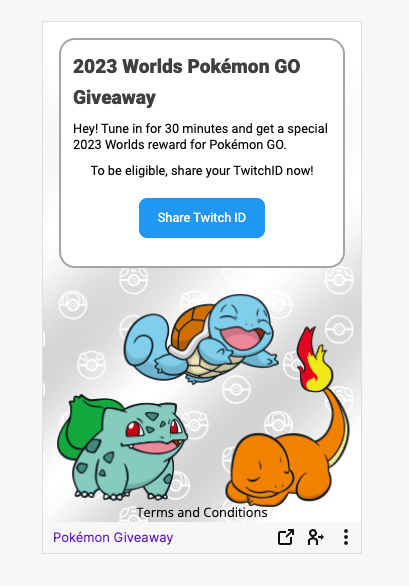This is a screenshot from an application associated with The Pokémon Company and featuring Twitch integration. The primary display is mostly white, with a central box containing dark grey text titled "2023 World's Pokémon Go Giveaway." The text invites users to tune in for 30 minutes to receive a special 2023 World's reward for Pokémon Go, and suggests sharing their Twitch ID to be eligible. Below the text, there is a blue and white button labeled "Share Twitch ID."

The background behind this central box is a subtle grey and white pattern featuring various outlined Poké Balls, including Great Balls, Standard Poké Balls, Ultra Balls, and Master Balls. At the upper part of the screen, the joyful Pokémon Squirtle is depicted jumping and smiling. To the lower left, Bulbasaur is standing and smiling as well, looking to the left side of the screen. To the lower right, Charmander is illustrated with closed eyes, appearing to be peacefully sleeping.

Beneath these three Pokémon are the words "Terms and Conditions." Below that text, there is a white banner featuring the purple words "Pokémon Giveaway." Adjacent to this banner are several interactive buttons: one leading to follow the link to the site, a button with an icon of a person and an arrow, and three additional buttons for settings or menu options.